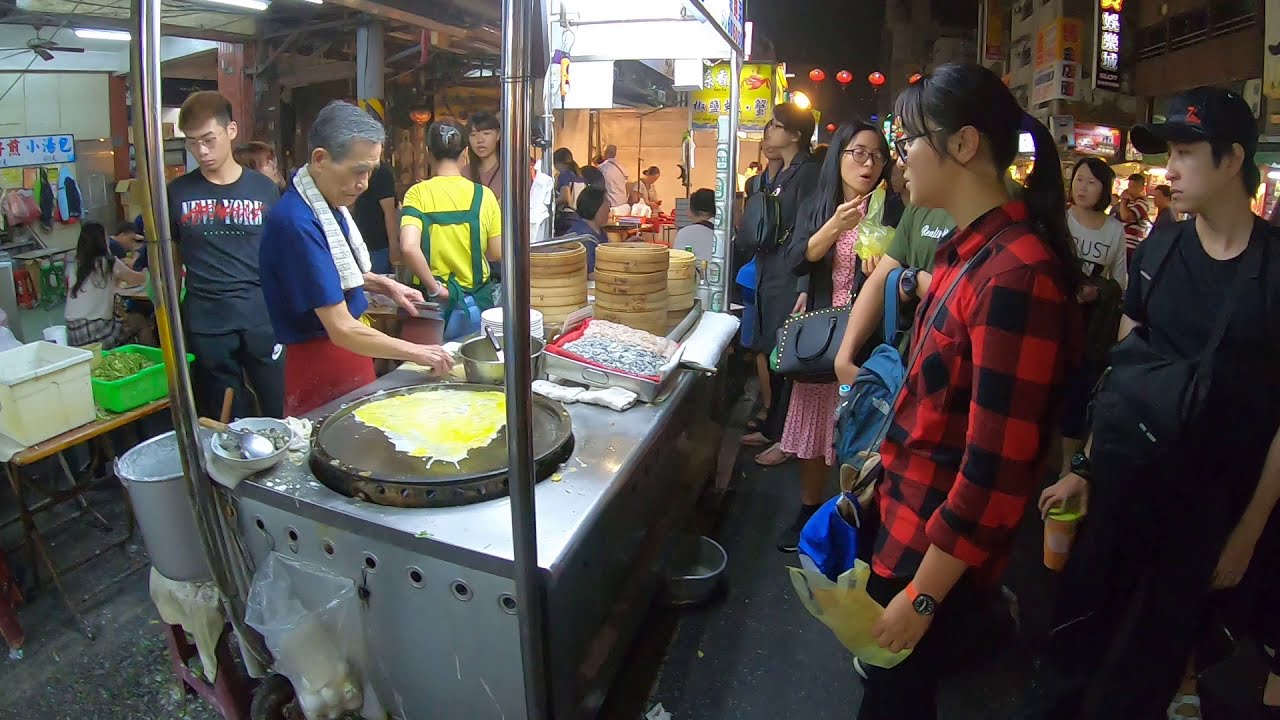In this nighttime street scene, a bustling crowd gathers around a lively food vendor. A young Asian woman with long brown hair, wearing glasses and a red and black plaid flannel shirt, stands to the right with a watch adorning her wrist. Behind her, a man dressed in black, including a black shirt and cap, holds a drink and wears a backpack. The focal point is a silver food cart where an Asian man, donning a blue shirt, red apron, and a towel around his neck, skillfully fries a large egg on a black wok. He also has a hairnet on. Next to him, a young boy with a "New York" t-shirt and glasses observes the scene. Various baskets, bags, and cans are scattered around the cart, which features bamboo shoot bowls and other cooking utensils. The atmosphere reflects the busy nightlife of a city street, with buildings silhouetted in the background and people eagerly waiting for their turn to buy food from the vendor.